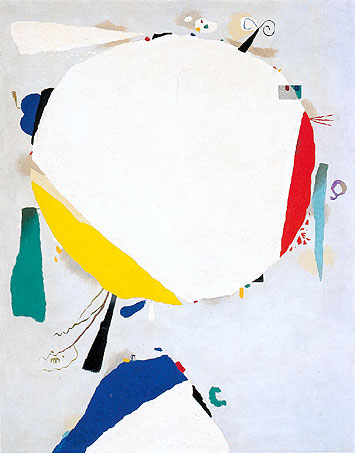This abstract mixed media artwork is set against a solid light gray background and is oriented in portrait format. Dominating the center of the composition is a large, predominantly white circle with torn paper edges, giving it a textured appearance. Slivers of this circle feature vivid yellow on the left and bold red on the right, with numerous fine black lines radiating outward. In the top left corner of the circle, a small black triangle with curving lines emerges, adding complexity to the composition.

Just above this circle, a light gray triangle subtly blends into the background, while below it lies a two-toned triangle. The bottom half of this lower triangle is white, and its top half is a striking blue. Surrounding the main elements, various torn paper strips—including colors like yellow, green, red, royal blue, and light blue—add layers and depth. Notable shapes and objects, including tree-like and boat-like forms, contribute to the intricate and dynamic nature of the painting.